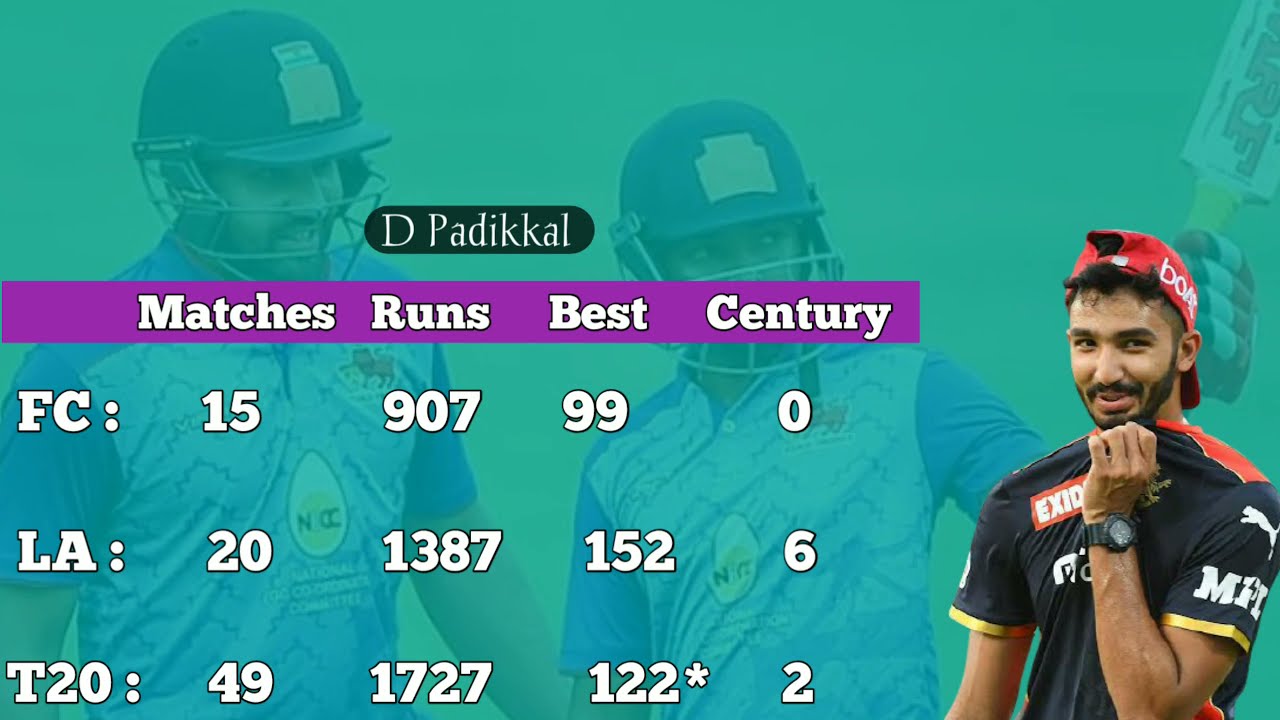This detailed image appears on a computer or television screen with a green background. At the center, there are two athletes with a blue film tint overlay, wearing protective batting helmets and light-colored jerseys with darker sleeves. The helmets have a unique symbol resembling a square with a little rectangle on top. The athletes, slightly blurred like a watermark, are positioned to the left and middle, looking to the right. One seems to be holding a stick, possibly a lacrosse stick, with gloves on.

In the lower right corner, there’s a man in a distinct, vivid portrayal. He has a backwards-facing red baseball cap, a blue shirt adorned with various boxed logos, including one resembling a little puma or panther near a red stripe on his left shoulder, and possibly letters like M, I, or MIT nearby. He possesses a mustache and beard and is seen contemplatively resting his hand, which sports a black watch, on his chin, gazing slightly to the left.

Overlaying these visuals, statistical details are prominently displayed. At the top, it reads "D. Padikkal." Below it, separate sections list stats such as "Matches: 15, Runs: 907, Best: 99, Century: 0" and further include categories labeled FC, LA, and T20, suggesting cricket game statistics. The information appears cleanly in white text on a black background, with a purple box highlighting terms like "matches, runs, best in century."